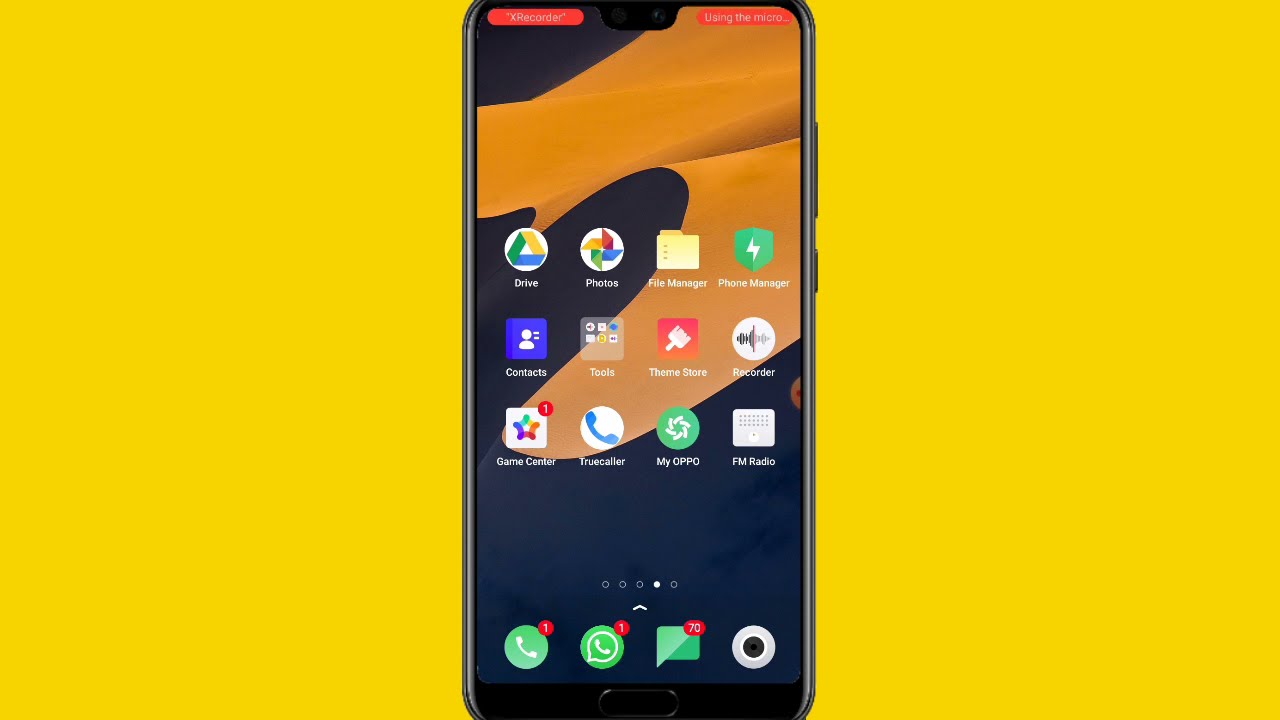This image depicts a black mobile phone centered on a bright yellow or orange background. The phone's screen features a black background with light brown or orange waves. The home screen is organized into rows of app icons, with four icons per row and three rows in the middle of the screen. The listed apps include Game Center, True Caller, My OPPO, FM Radio, Recorder, Theme Store, Tools, Contacts, Google Drive, Google Photos, File Manager, and Phone Manager. At the very top left, a small red rectangle with "X Recorder" is visible, and in the top right, some text reads "using the micro."

At the screen's base, five open white circles indicate pagination, with the fourth circle being filled. Below these circles are four larger icons: a green phone icon with one notification, a teal WhatsApp icon, another teal icon possibly for email with an old-fashioned design and ten notifications, and finally, a white camera icon. Additionally, the voicemail icon on the home screen has one notification. The intricate details and color contrasts create a visually engaging and informative image of a mobile phone's interface.